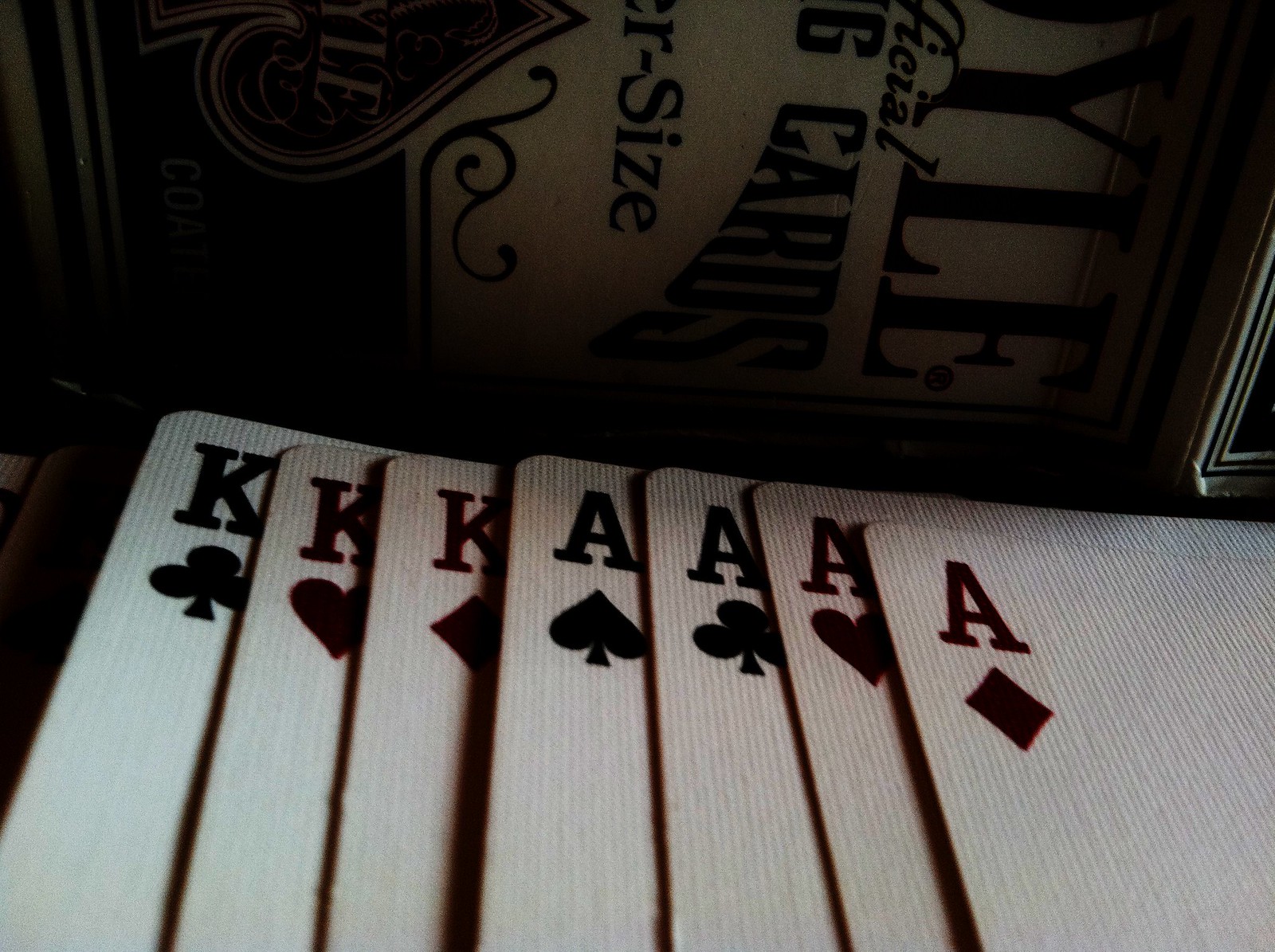The image features a collection of playing cards prominently displayed at the forefront. These cards appear aged, with a background reminiscent of a sun-faded, tightly-packed white picket fence gradually turning brown. Among the cards, there are three Kings (King of Hearts, King of Diamonds, and King of Clubs) and all four Aces (Hearts, Diamonds, Clubs, and Spades). Interestingly, all the suits, including those traditionally red (Hearts and Diamonds), are rendered in black. 

In the background, a box, seemingly meant to store the cards, lies on its side. The partially visible text on the box reads "YLE," likely referring to the brand Royale, known for its playing cards, and includes phrases like "special cards" and "size," although the full text is obscured. The image, slightly off in color representation, suggests the possibility of it being AI-generated, given the unusual coloring of the suits.